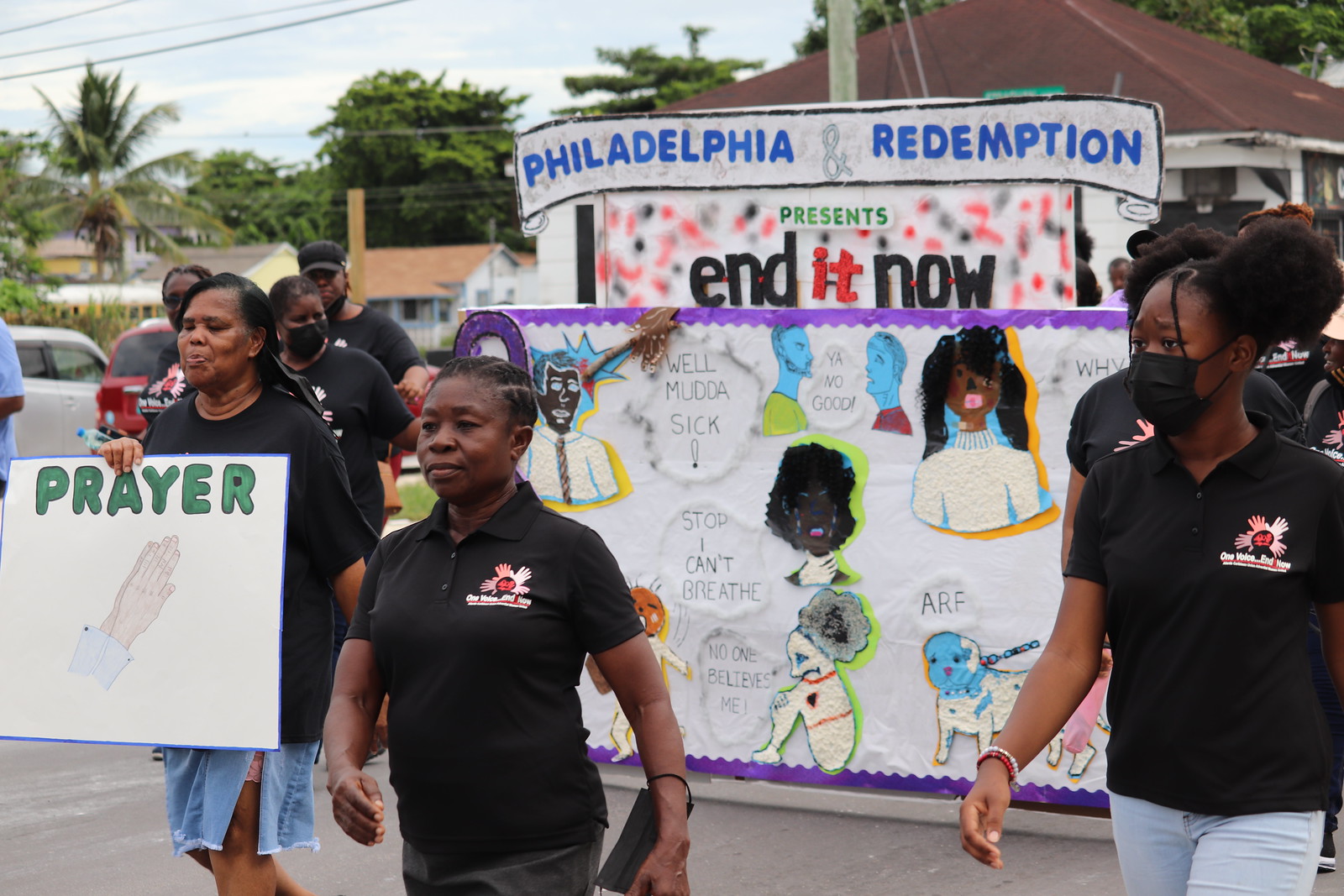In this detailed outdoor daytime scene, a group of predominantly African-American people is captured marching in support of preventing violence against people. They are all dressed in black shirts, each featuring an unreadable logo on the left chest, paired with various bottoms. Some participants are wearing face masks. The diverse group includes a woman on the left holding a green sign with praying hands, labeled "prayer." In the background, a prominent float displays signs and slogans, including "Philadelphia and Redemption presents End It Now," along with a border of purple surrounding photos and statements like "No one believes me," "I can't breathe," and "Stop." The setting includes a sky dotted with palm and green trees, suggesting a possibly warmer locale. The image not only captures the immediate marchers and their handmade signs, but also hints at more participants and city buildings just beyond the frame.